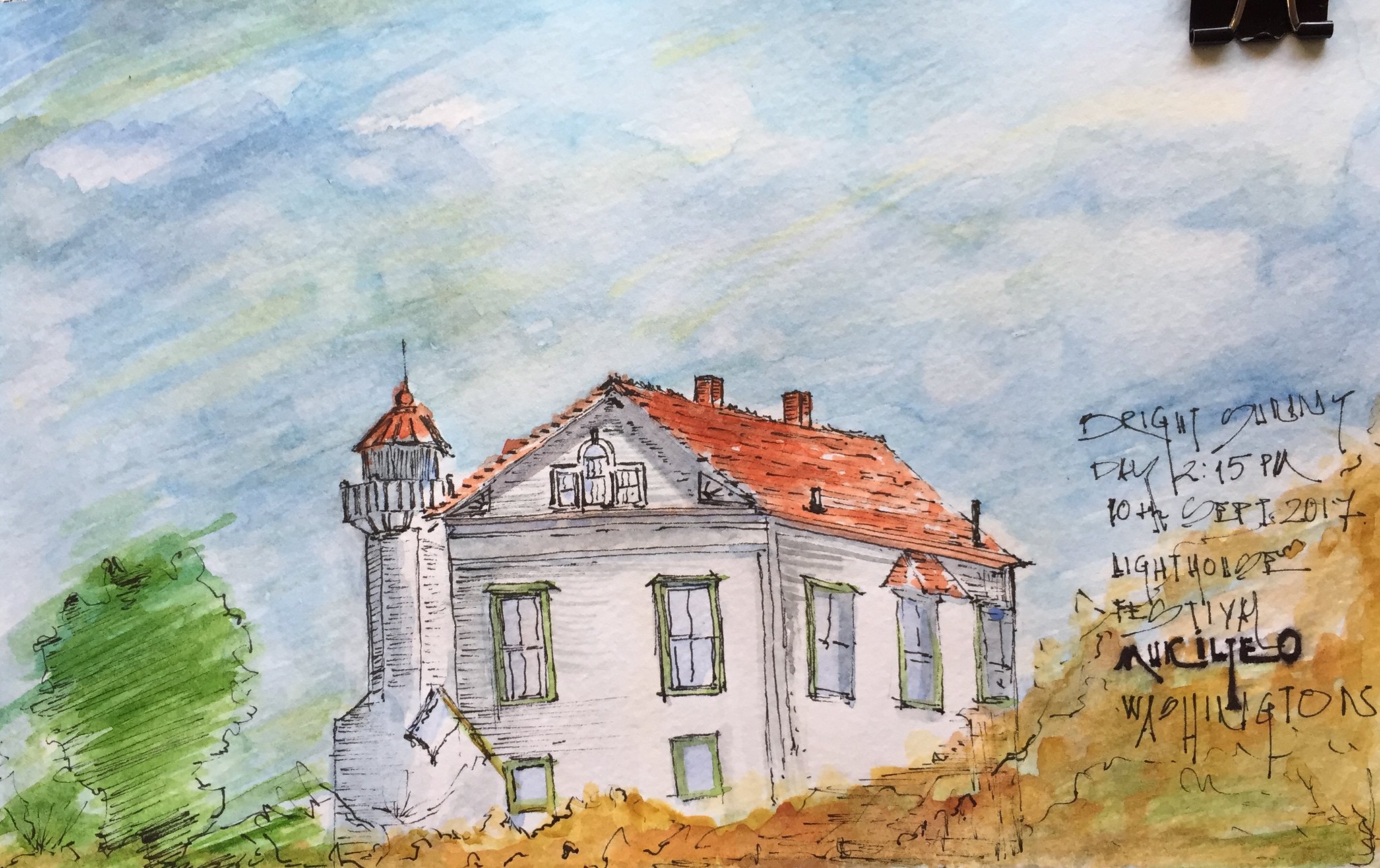This intricate watercolor painting, accentuated with dark pen highlights, beautifully captures a serene hillside scene. Dominating the composition is a stately white lighthouse tower, detailed with gray highlights and black accents, standing proudly beside a large white house. Both structures feature charming brown thatched roofs, adding a rustic touch to the scene. The hillside, rendered in warm shades of brown, complements the buildings and creates a harmonious palette. Lush greenery peeks through in the lower left corner, adding a splash of nature's vibrancy. The sky above is a mix of streaked blues with subtle hints of green, evoking a tranquil, breezy day. Intriguing but illegible pencil and pen sketches of words and numbers in the lower right corner add a mysterious element, inviting viewers to ponder their meaning.